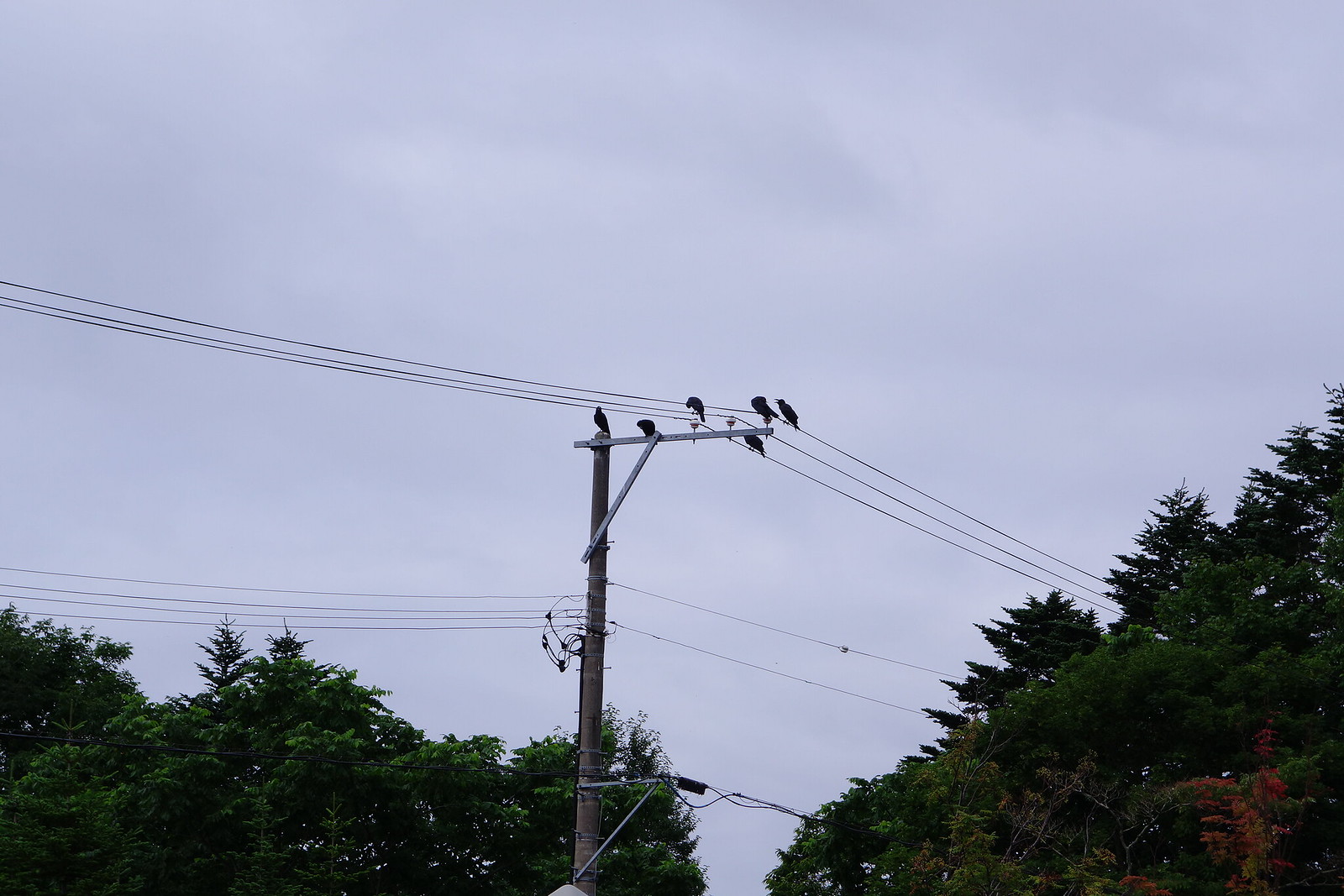The photograph captures a wooden electricity pole standing against a light blue, overcast sky. The sky is filled with diffuse clouds, suggesting dimmed sunlight. Perched atop the pole and its extending cables are six small black birds, likely crows, with their black feathers contrasting sharply against the muted sky. The birds are perched on two rows of black electric cables that span horizontally across the image, with some birds facing front and others in profile. At the bottom left and right corners, large, dense green trees with some autumn-red foliage intrude into the frame, their luxuriant leaves filling much of the lower part of the image. The composition centers on the verticality of the wooden pole and the horizontal stretch of the cables, capturing a tranquil moment of nature intersecting with human-made structures.